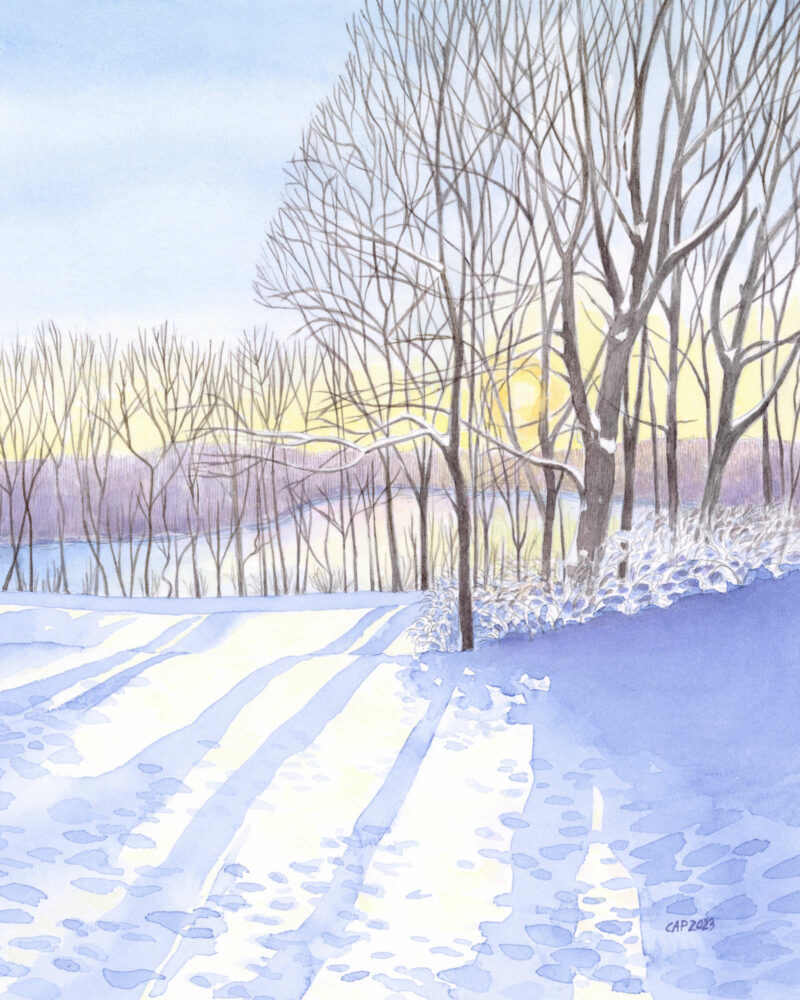This image is a serene and peaceful painting of a snowy landscape rendered in watercolor. The scene is outdoors during winter, indicated by the snow-covered ground and leafless trees. In the foreground, there's a wide expanse of snow with long, blue-tinted shadows cast by the trees, which some of them look like they have snow resting on their bare branches. Towards the right side of the painting, the shadows almost completely cover the snow. Near the bottom of the image, there are patterns in the snow that resemble footprints or dappled light. 

In the middle of the painting, a row of tall, slender trees without leaves extends across the landscape, while more trees can be seen farther back, adding depth to the scene. Behind these trees lies a hazy, indistinct mountain range or possibly more trees blending into the background. 

The sky above transitions from a soft yellow glow near the horizon, suggesting an early morning sunrise, to a light blue with thin, white cirrus clouds. This yellow strip and blue sky above it add warmth and brightness to the chilly scene. The painting, presented in a vertical rectangle without a frame, is signed with "Cap 2023" at the bottom.